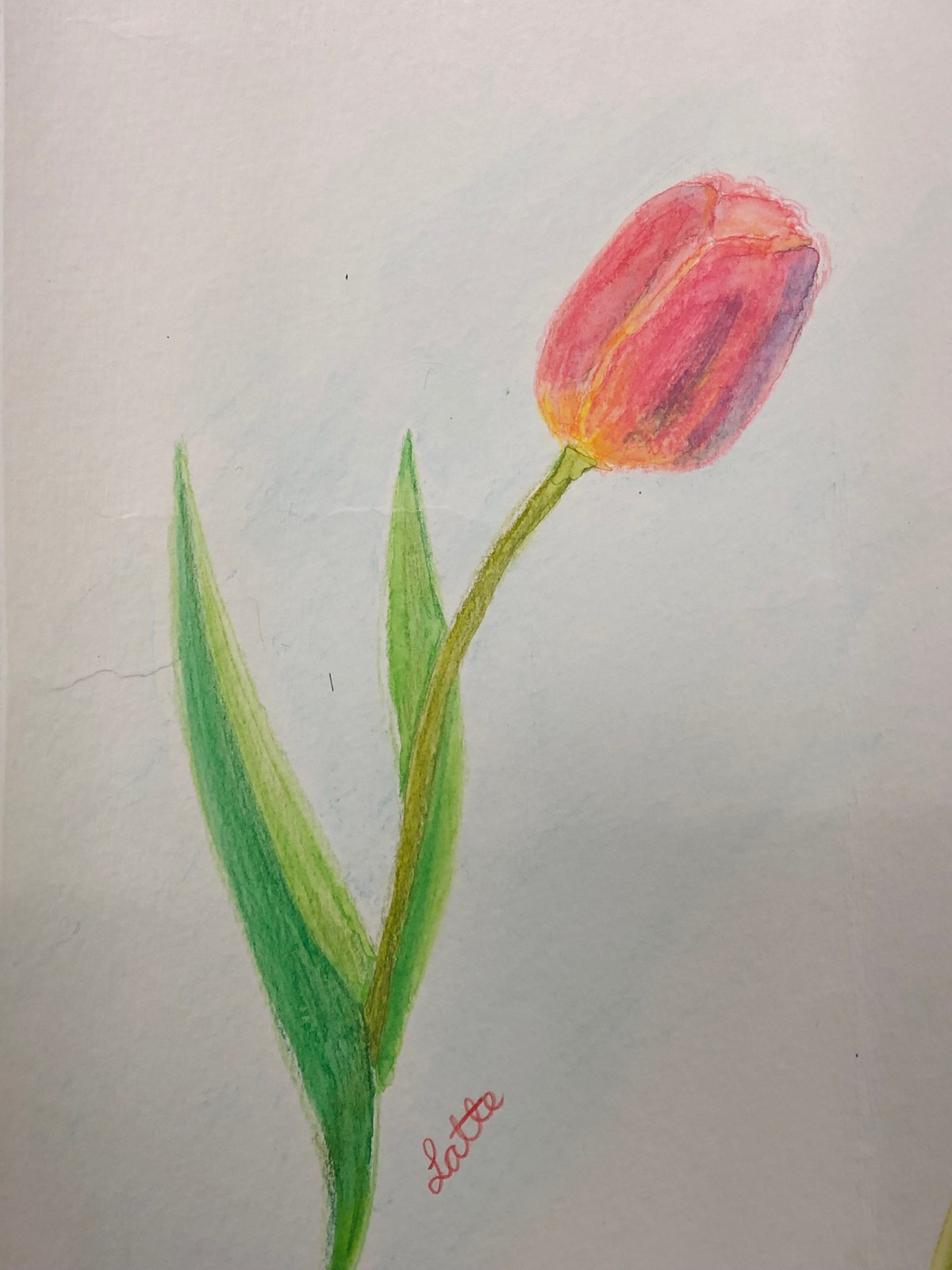The artwork showcases a vibrant tulip rendered in a combination of colored pencils and possibly crayons. The tulip features a striking bloom with petals blending shades of pink, lavender, and orange, creating a lively and dynamic bud. Its sturdy stem supports vertical leaves that extend gracefully down to the bottom of the composition, which is set against a light gray, off-white background. The flower appears to have been meticulously outlined in pencil before being filled in with rich color, adding depth and texture to the piece. At the bottom of the page, beside the tulip, the artist's signature, "LATTE," is delicately inscribed, affirming the creator's identity. This detailed depiction highlights the beauty of the tulip, making it the focal point of the light gray canvas.